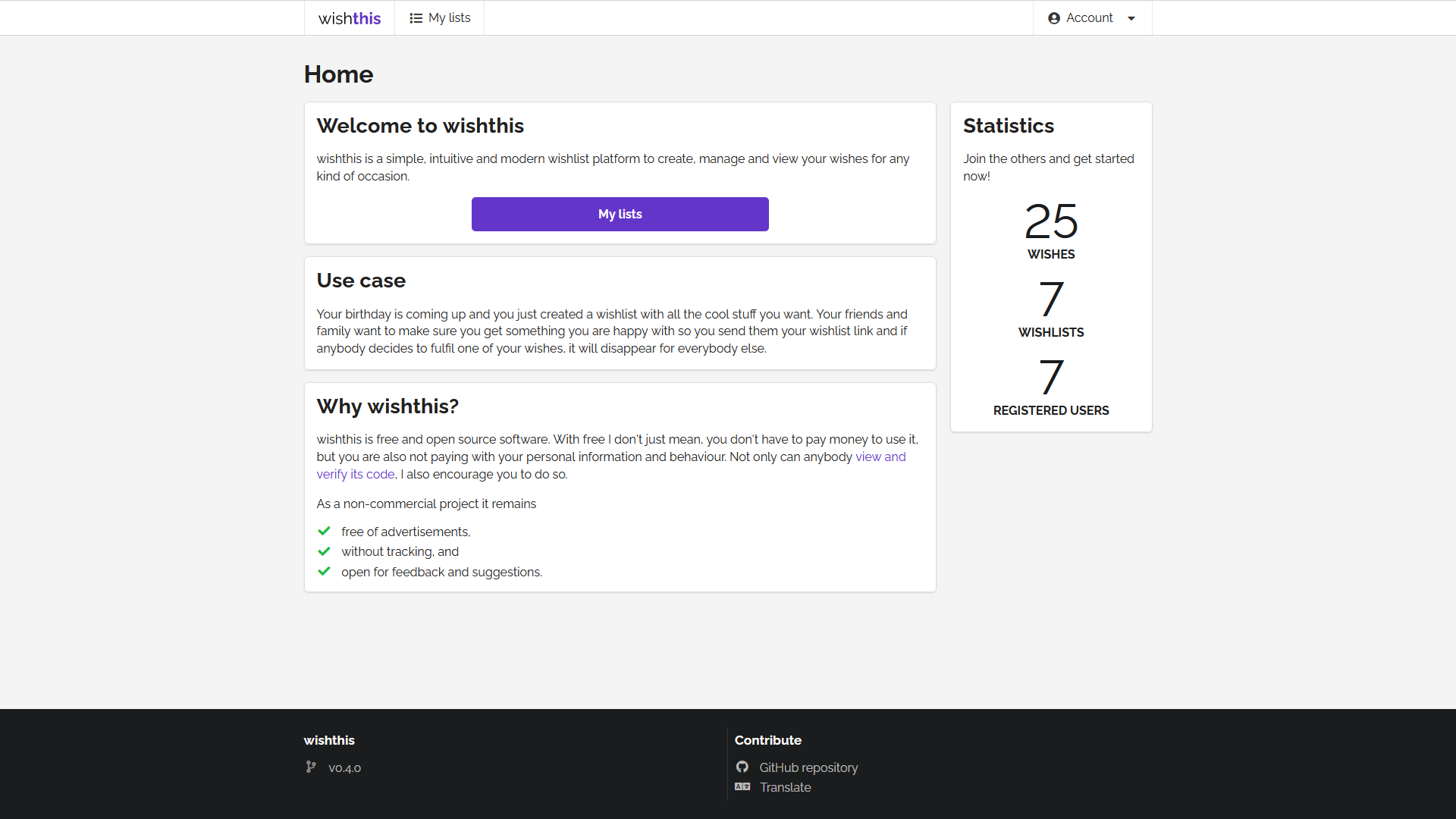This is a detailed description of the "Wish This" web page:

At the top of the screen, occupying roughly one-twentieth of the vertical space, there is a section with a white background. Below this, taking up approximately three-quarters of the lower part of the screen, there is a large gray rectangle. Beneath this gray section is a black rectangle featuring links to other sites, including options to translate the webpage. 

In the center of the web page, the text reads "Home. Welcome to Wish This." This message introduces "Wish This" as a simplistic, intuitive, and modern platform designed for creating, managing, and viewing wishes for any occasion. 

Further down the page, in a purple hyperlink, there is a navigation link labeled "My Lists." Below this link, the text describes various use cases, such as organizing birthday presents or selecting gifts for someone, emphasizing that once a wish is fulfilled on the site, it disappears for others to prevent duplications.

Continuing further, the site explains the benefits of using "Wish This." Notably, it is a free and open-source platform, meaning users do not need to spend any money to access its features. Additionally, it is a non-commercial project free from advertisements and user tracking, and it welcomes feedback and suggestions.

On the right side of the page, there is a rectangular section displaying the site’s statistics, which include: 25 wishes, 7 wish lists, and 7 registered users.